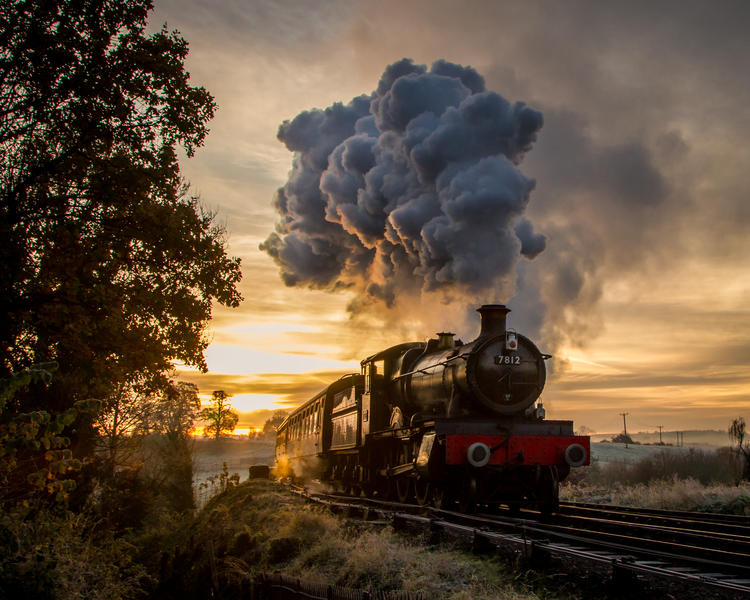In this dramatic twilight photograph, an old-fashioned steam train, numbered 7812 in white letters, charges down the tracks beneath a dark, cloudy sky. The red front of the train, crowned with a chimney billowing a thick, dark plume of smoke, commands attention as it emerges from under a bridge. Positioned from a vantage point to the left of the tracks, the image captures the train’s powerful advance from the lower center, trailing carriages behind. The scene is framed by a tall tree rising on the left, with additional trees and grassy areas adorning the countryside. The setting sun casts a warm, golden hue low on the horizon, providing a striking contrast to the moody, cloud-covered sky. This captivating blend of nature and machinery presents a nostalgic yet dynamic scene of a bygone era.